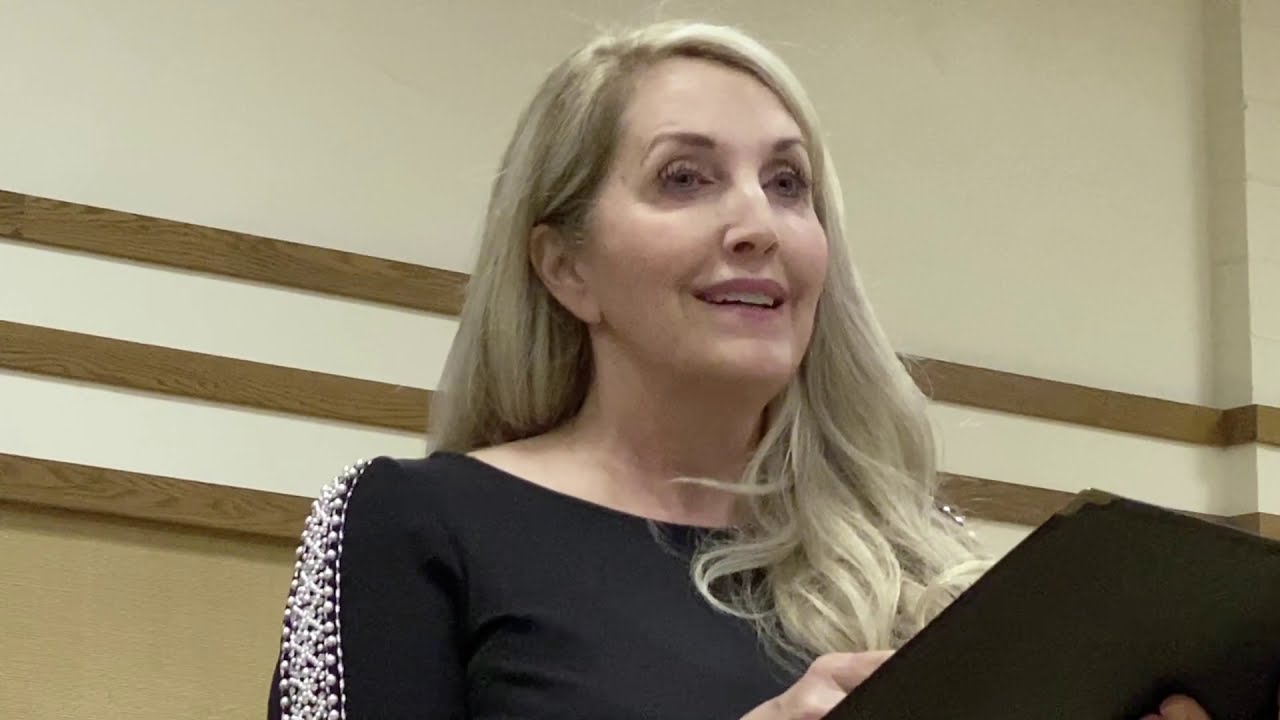In the photo, an older Caucasian woman is captured from a slightly below angle, making her look as if she's giving a presentation or speech. She has very fair skin and light blonde, almost bleach-blonde hair. Her hair falls in soft waves and curls, draped behind her left ear and cascading over her right shoulder. She has dark brown, arched eyebrows and is wearing makeup with long eyelashes, her mouth slightly open as if speaking. Dressed in a black dress with a high neck, the intricate design features ornate pearly white beads running in a stripe pattern from her shoulders down to her sleeves. In her hands, she holds a black binder or folder, appearing prepared to read from or reference it. The background reveals that she is inside, standing in front of a well-lit white wall accented with three horizontal wooden stripes and a beige lower section. This close-up head and shoulder shot gives a detailed view of her expression and attire, emphasizing her poised and confident demeanor.